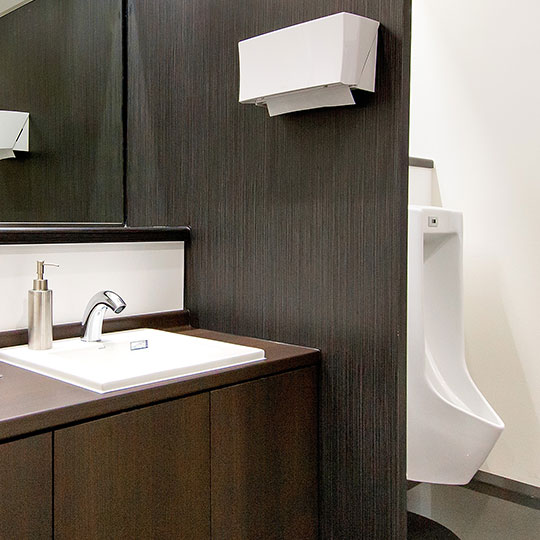The image depicts a modern men's bathroom with a distinct layout. On the right side, there's a white urinal mounted on a light-colored wall with speckled brown tiles below it. The urinal area is partially separated by a dark brown wooden partition. Above the partition, there’s a white rectangular paper towel holder with a bit of paper towel sticking out. 

Dominating the left side of the image is the sink area. The brown cabinet below supports a white square porcelain sink fitted with a chrome faucet. Beside the sink is a gold-colored, pump-style soap dispenser. Above the sink, there's a mirror and a ledge, providing space for small items. The walls and countertops feature a wood grain pattern, enhancing the modern look of the bathroom. The dark gray walls and speckled brown tile flooring contribute to the contemporary aesthetic as well.